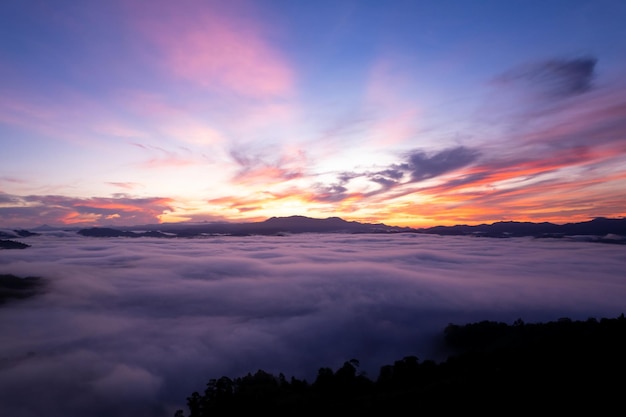This photograph captures a breathtaking sunset taken from a high elevation, presenting a view above the clouds. The scene features a stunning gradient sky where the upper portion transitions from a bright blue to radiant shades of pink and purple. Dominating the horizon, the sun emits golden and orange rays that gently disperse across the sky. In the center of the image, a sea of clouds stretches out, appearing white and flat, punctuated by darker cloud formations near the horizon. Below, in the right-hand corner, the tops of trees are visible, hinting at a lofty viewpoint. Across the middle distance, the silhouettes of mountain peaks emerge, adding depth and character to the landscape. The overall composition beautifully captures the serene and majestic interplay of light, color, and elevation.